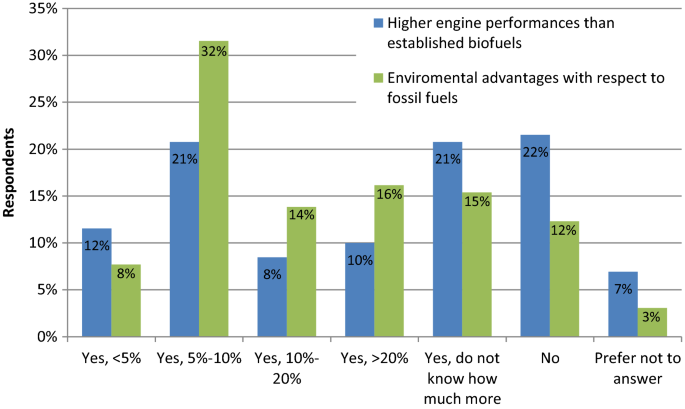The image shows a detailed bar graph with a horizontal background of gray or black and gray lines. On the left side of the graph, a vertical axis is labeled "respondents" with percentages marked in increments of 5%, ranging from 0% to 35%. At the top of the graph, a legend specifies that blue bars represent "higher engine performance than established biofuels" and green bars represent "environmental advantages with respect to fossil fuels." 

Each section of the graph has two vertical bars; the blue bar on the left and the green bar on the right. Below the graph, text segments span horizontally, each with varying percentage ranges. The categories include "yes" under 5%, "yes" at 5%-10%, "yes" at 10%-20%, "yes" at 20%, "do not know how much more," and "prefer not to answer."
 
Detailed percentages for each category:
- Under 5%: Blue at 12% and Green at 8%.
- 5%-10%: Blue at 21% and Green at 32%.
- 10%-20%: Blue at 8% and Green at 14%.
- 20%: Blue at 10% and Green at 16%.
- Do not know how much more: Blue at 21% and Green at 15%.
- Prefer not to answer: Blue at 22% and Green at 12%.
- Additional category: Blue at 7% and Green at 3%.

All figures and text are in black, and the sequential arrangement highlights the survey results regarding perceptions of engine performance and environmental advantages of biofuels compared to fossil fuels.